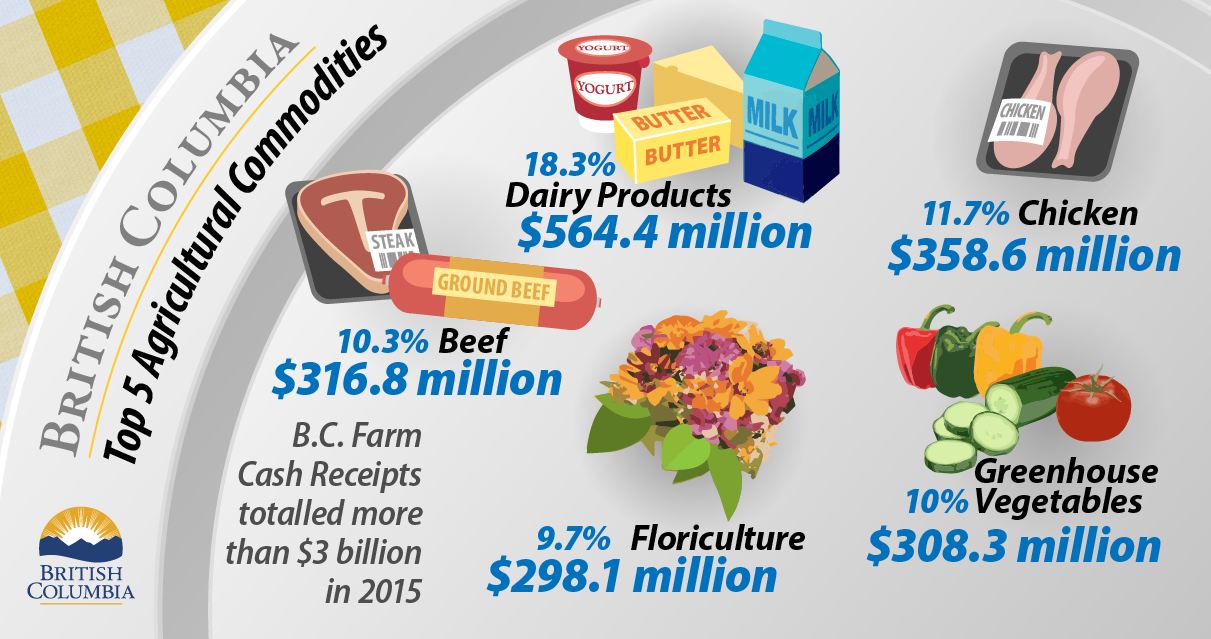The image showcases a colorful and informative depiction of British Columbia's top five agricultural commodities, displayed in a whimsical clip art style. Centered on the image is a white plate set against a yellow-and-white picnic blanket backdrop. The plate prominently features the British Columbia insignia, with a sun rising over mountains and the text "British Columbia" written in gray. Above the logo, the title "Top Five Agricultural Commodities" is displayed in bold black print. 

The commodities are illustrated around the plate with corresponding percentages and monetary values from 2015:

- **Beef**: Depicted with a steak wrapped in packaging, representing 10.3% of the total, worth $316.8 million.
- **Dairy Products**: Shown with images of butter, milk, and yogurt, accounting for 18.3%, worth $564.4 million.
- **Floriculture**: Illustrated with colorful flowers, making up 9.7%, valued at $298.1 million.
- **Chicken**: Displayed as a package of raw chicken wings, comprising 11.7%, worth $358.6 million.
- **Greenhouse Vegetables**: Depicted with a sliced cucumber, peppers, and a tomato, representing 10%, valued at $308.3 million.

The entire image highlights that BC farm cash receipts totaled more than $3 billion in 2015, combining the agricultural economic contributions in a visually engaging manner.